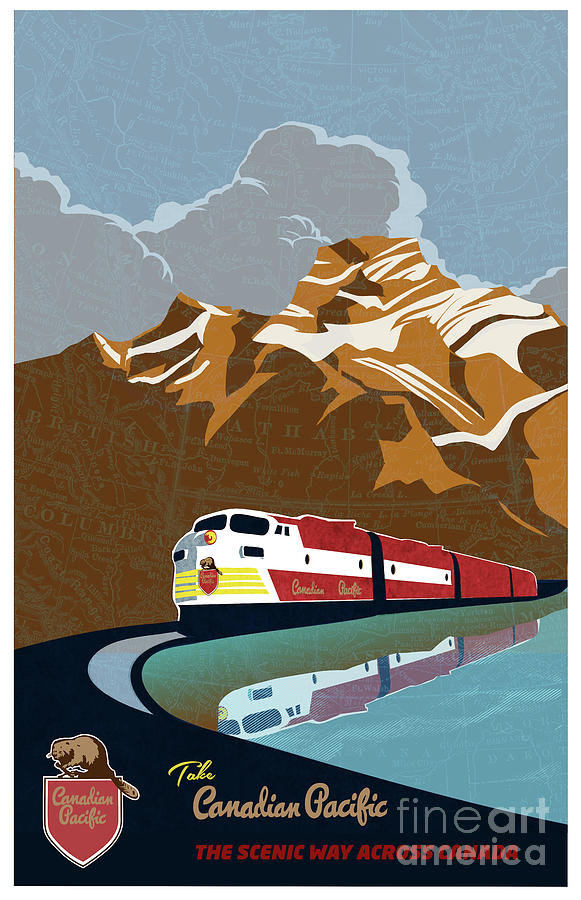This detailed art poster, likely created using a graphic design program such as Photoshop, promotes the Canadian Pacific Railway with an artistic blend of digital illustration and subtle map data. Dominating the center is a striking image of a red and white diesel locomotive, comprised of a yellow-grilled engine and three following cars, journeying along a train track beside a reflective lake. The locomotive's design features a prominent white stripe flanked by red coloring, with the two rearmost cars being solid red.

Above the train, a majestic brown-orange mountain, seemingly embedded with subtle map details of British Columbia, rises against a backdrop of dark clouds and a soft blue sky. The photograph subtly integrates various map elements into the scenery, creating a textured, layered effect.

At the bottom of the poster, the slogan "Take Canadian Pacific, the scenic way across Canada" is prominently displayed in the center, inviting viewers to embark on a picturesque journey. Flanking this slogan, the Canadian Pacific logo featuring a beaver appears on the lower left, and a Fine Art America watermark is placed on the lower right. The combination of these elements creates a visually appealing and informative advertisement for the Canadian Pacific Railway.